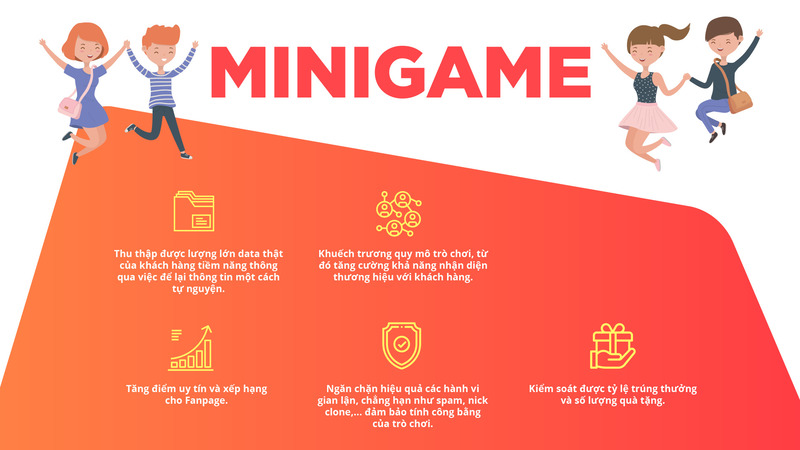The image features a central heading in bold, all-caps red letters reading "MINIGAME" against a white background. Flanking this heading are cartoon-style characters: to the left, a red-headed boy and girl wearing blue, and to the right, a brunette boy and girl. All are depicted joyfully jumping and holding hands. Beneath them is an asymmetrical shape that transitions from orange to red. Within this colorful section are five distinct yellow logos, each accompanied by white text in an unreadable foreign language. The logos include, from left to right: stacked floppy disks, four connected circles with person outlines, a bar graph with an ascending arrow, a badge with a check mark, and a hand holding a gift. The background of the entire ad is a lightish red, enhancing the vibrant and playful nature of the visual overall.